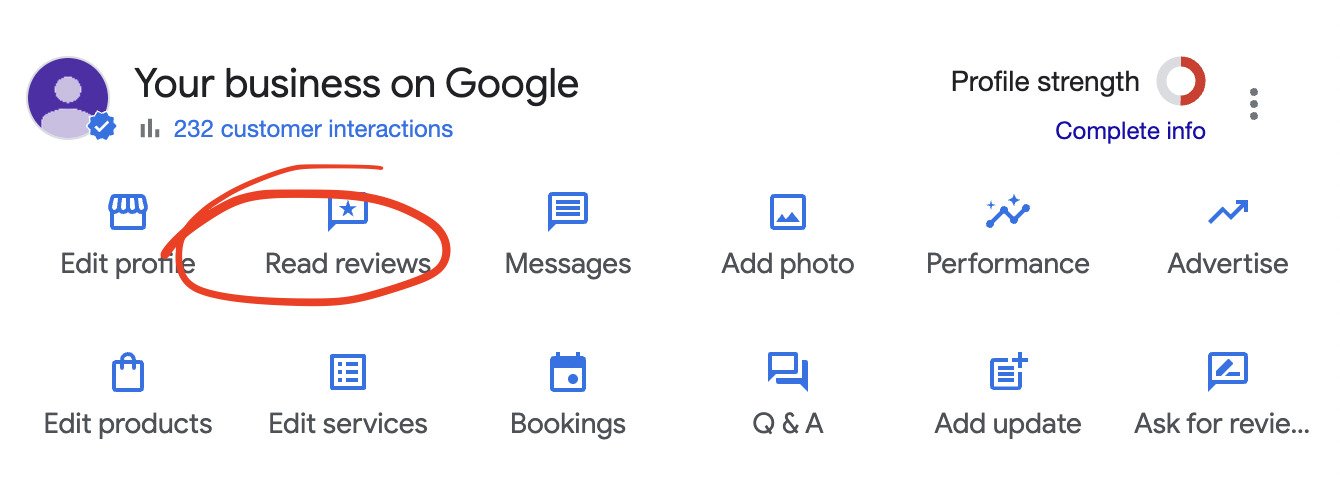The image features a white background with various elements related to managing a Google business profile. In the upper left corner, there's a light purple icon associated with a profile, accompanied by the text "Your business on Google" in black font. Below this, it's noted that there have been "232 customer interactions" under the same heading. 

To the right, there's a section showing the "Profile Strength" indicator, which comprises a circular outline that is half-red and half-gray. Below this circular indicator, the text "Complete Info" appears in blue. To the right of these elements, there are three vertical dots, signifying additional options.

In the center of the image, there's a grid of six icons arranged in two rows, each icon accompanied by a label in black font and a blue symbol:
- Edit profile
- Read reviews (this option is circled)
- Messages
- Add photo
- Performance
- Advertise

The second row contains:
- Edit products
- Edit services
- Bookings
- Q&A
- Update
- Ask for reviews (the text for this extends beyond the visible area, marked with "dot dot dot")

The predominant colors in the image are purple, light purple, black, blue, gray, white, and red. Each option has a corresponding blue icon, while all text is rendered in black. There is no visible border surrounding any elements.

Overall, the image appears to be a screenshot or interface related to managing specific functions and viewing statistics for a Google business profile.